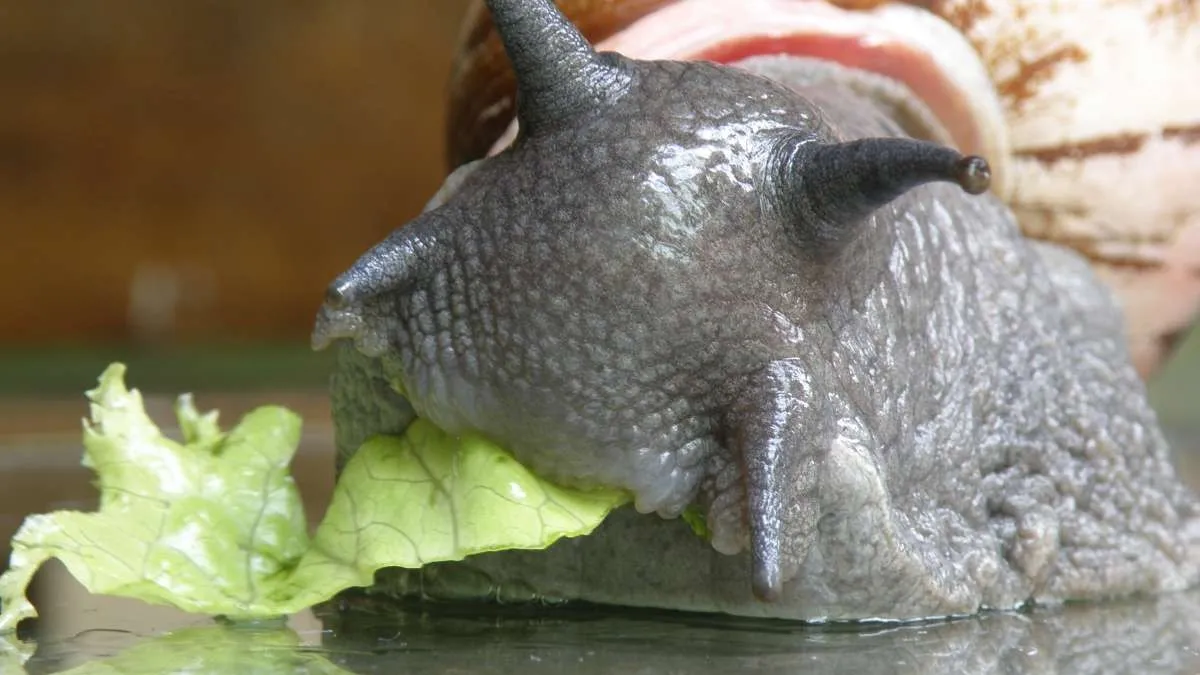This is a close-up photograph of a very large grey snail, prominently featuring its head as it eats a piece of bright green lettuce. The snail's skin is textured with varying shades of grey, interspersed with small, raised, lighter grey areas. The snail's eyes, located on two small, tentacle-like horns, are visible on either side of its head. Its mouth is a solid grey line, where a strip of green lettuce dangles down onto a reflective, shiny grey surface. The snail is partially extended from its shell, which is positioned diagonally from the center up to the top right of the image. The shell is a cream color with dark brown lines near the head area and has a raised lip that runs across the back of the snail’s head. The background is blurred with shades of brown and a hint of green, ensuring the viewer’s focus remains on the front of the snail.